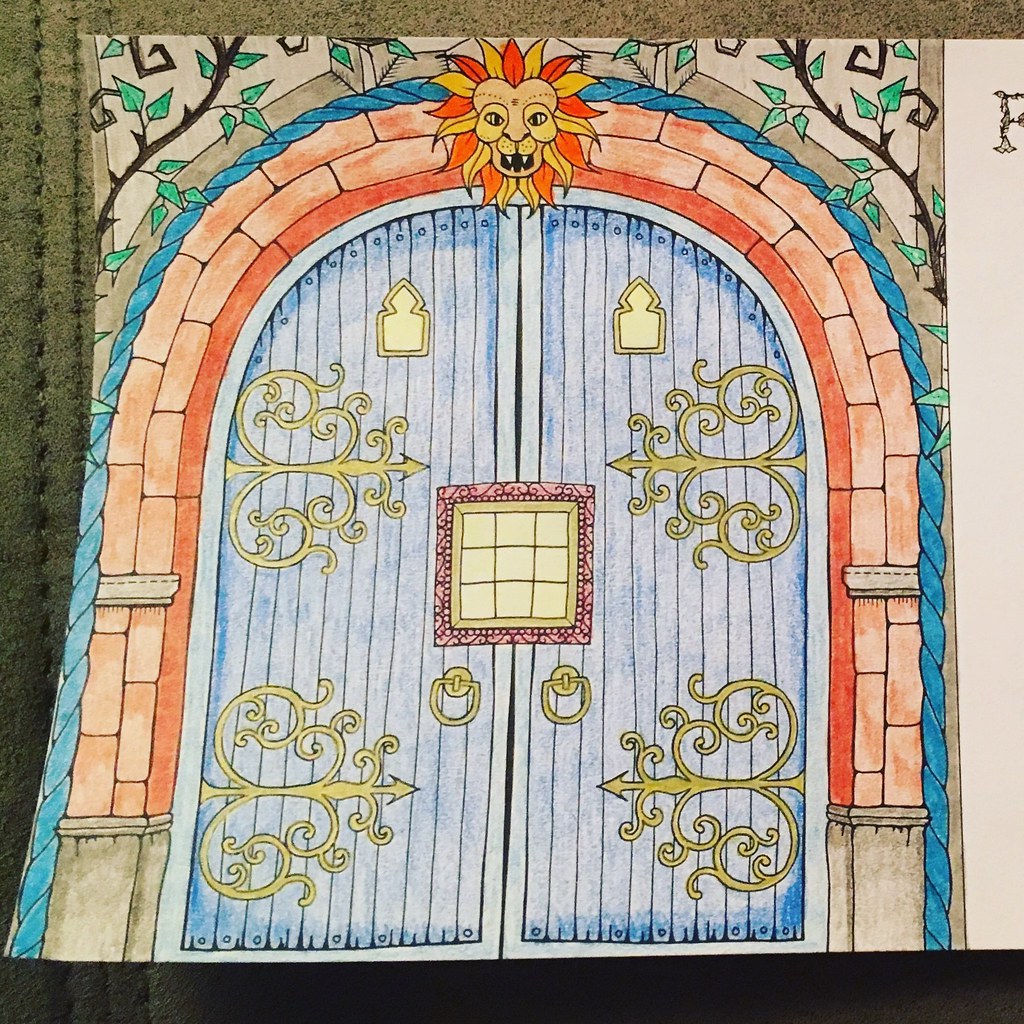The image is a highly detailed colored pencil drawing of a castle-like, ornate doorway. The large, wooden door, painted in a light blue hue and composed of planks, features elaborate gold adornments, including two brass knockers. The door opens from the middle, and at the top of the arch is a prominently detailed lion's head in orange-yellow, with its mouth open, showcasing its teeth. Surrounding the doorway is a brick border made up of predominantly red and light red stones, arranged in a layered pattern. The archway itself is crafted with a mix of red and orange stones, forming a bullet-like shape. Additional intricate designs and a square grid outlined in red swirls can be seen on the door, adding to its ornate appearance. The entire drawing is presented on a piece of paper, with an "F" faintly visible in the top right-hand corner, alluding to the artist's initials. The artwork lacks an artist's name but stands out for its intricate detail and vivid coloring.